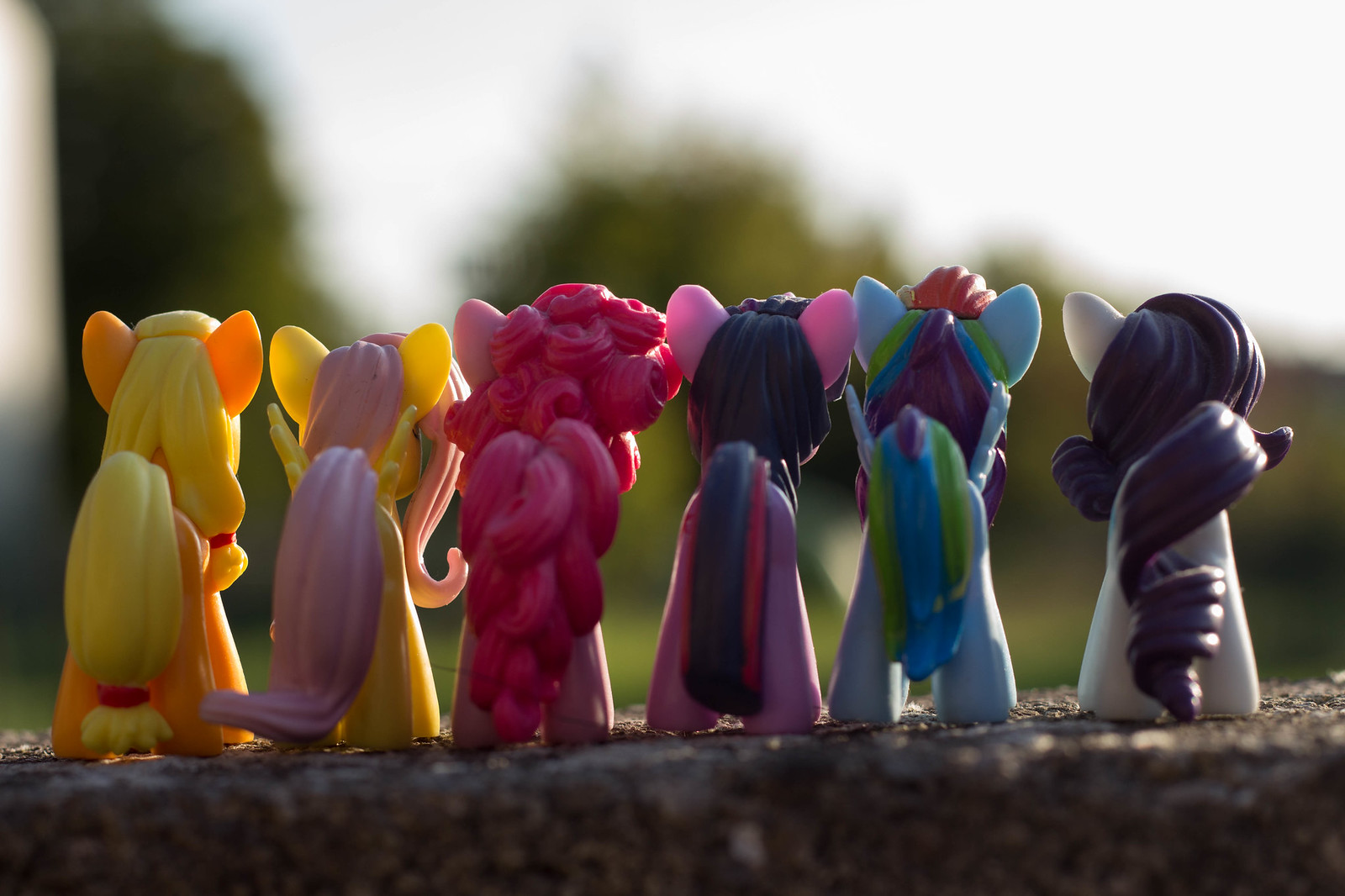The image depicts six My Little Pony figurines lined up in a row, each one facing away from the camera and looking out over a blurred landscape. The ponies are positioned on an outdoor, somewhat uneven surface that might be dirt or rocks. The background shows a lawn with trees in the distance under a gray, hazy sky. The first pony on the left is yellow with orange ears and red hair ties. Next to it is a pink pony with yellow hair. The third pony is very pink with curly hair in two shades of pink. The fourth pony is purple with a navy blue and red tail. The fifth pony is blue with green, blue, and purple hair and tail, plus a hint of pink on its head. The last pony on the right side is light blue with a navy blue, swirled tail. All the ponies are facing outward, observing the distant landscape.